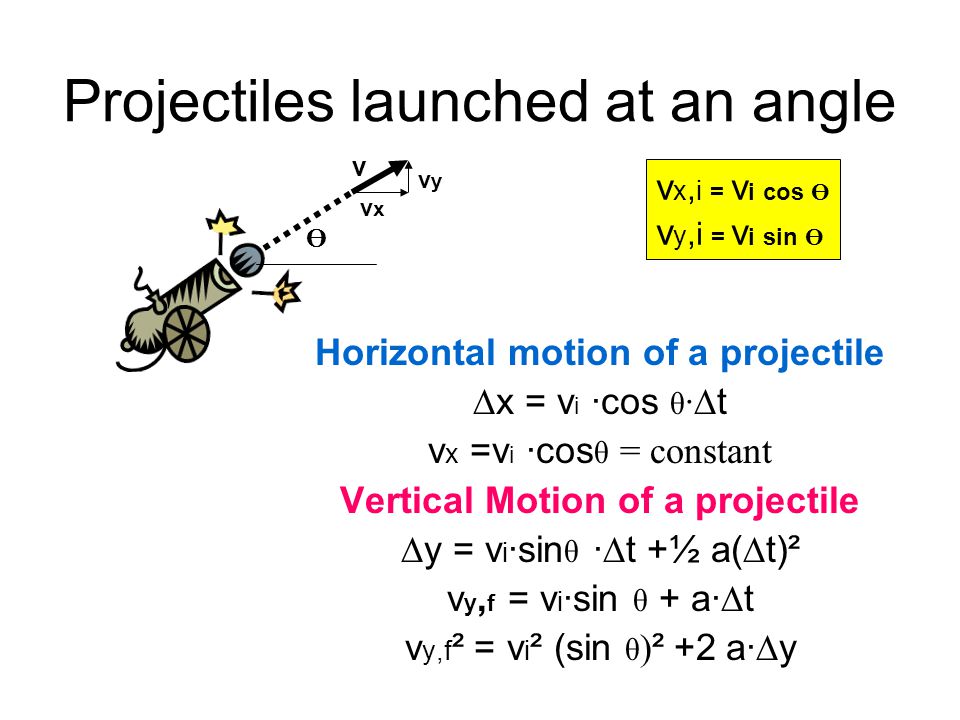The image, titled "Projectiles Launched at an Angle," illustrates the mathematical equations for both vertical and horizontal motion of a projectile. In the top-left corner, a cartoonish gray cannon is depicted firing a blue cannonball at an angle towards the northeast. Yellow stars with black stems adorn either side of the cannonball, which is followed by dotted trajectory lines and a dark arrow indicating its path. On the right side of the image, a prominent yellow box contains equations for the vertical and horizontal components of the projectile's motion, written in black text. Below the yellow box, the heading "Horizontal Motion of a Projectile" is displayed in blue, followed by its corresponding formula. Underneath this, the heading "Vertical Motion of a Projectile" appears in pink, with its associated formula written below in black text. The image seems to be an excerpt from a math textbook, showcasing how to calculate the motion of projectiles launched at an angle.